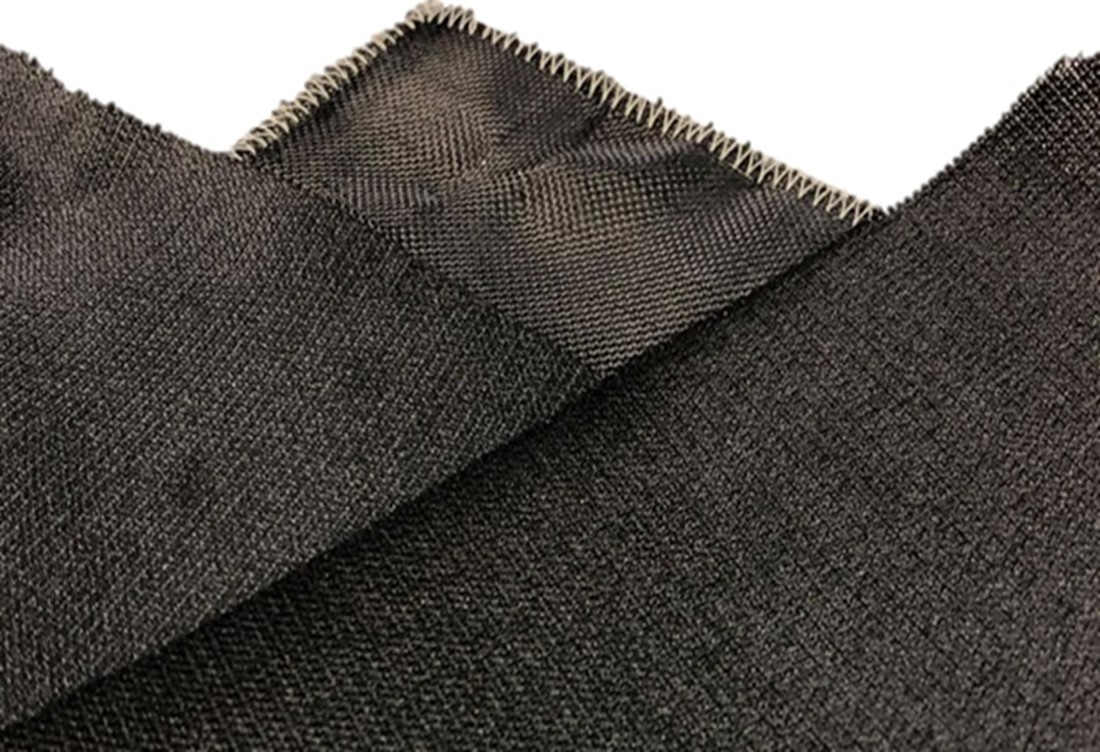This detailed close-up shot features several overlapping pieces of dark gray, charcoal-colored fabric with a coarse weave. The fabric covers most of the image, set against a white background at the very top. The overlapping arrangement is in a triangular fashion, revealing both the front and back sides of the material. The lower half, predominantly on the right side, exposes the texture of the front side, while in the upper middle portion, the back side of the fabric is visible. Notably, one piece showcases zigzagged tan-colored stitching running along its edges, suggesting a square or rectangular shape due to its perpendicular lines. The stitching detail, which has been serged with either white or tan thread, highlights the fabric's crafted edges. A segment on the left side also shows the front of the fabric, adding to the layered arrangement. The fabric includes a woven pattern with lighter gray and cream threads interspersed, reminiscent of upholstery fabric.